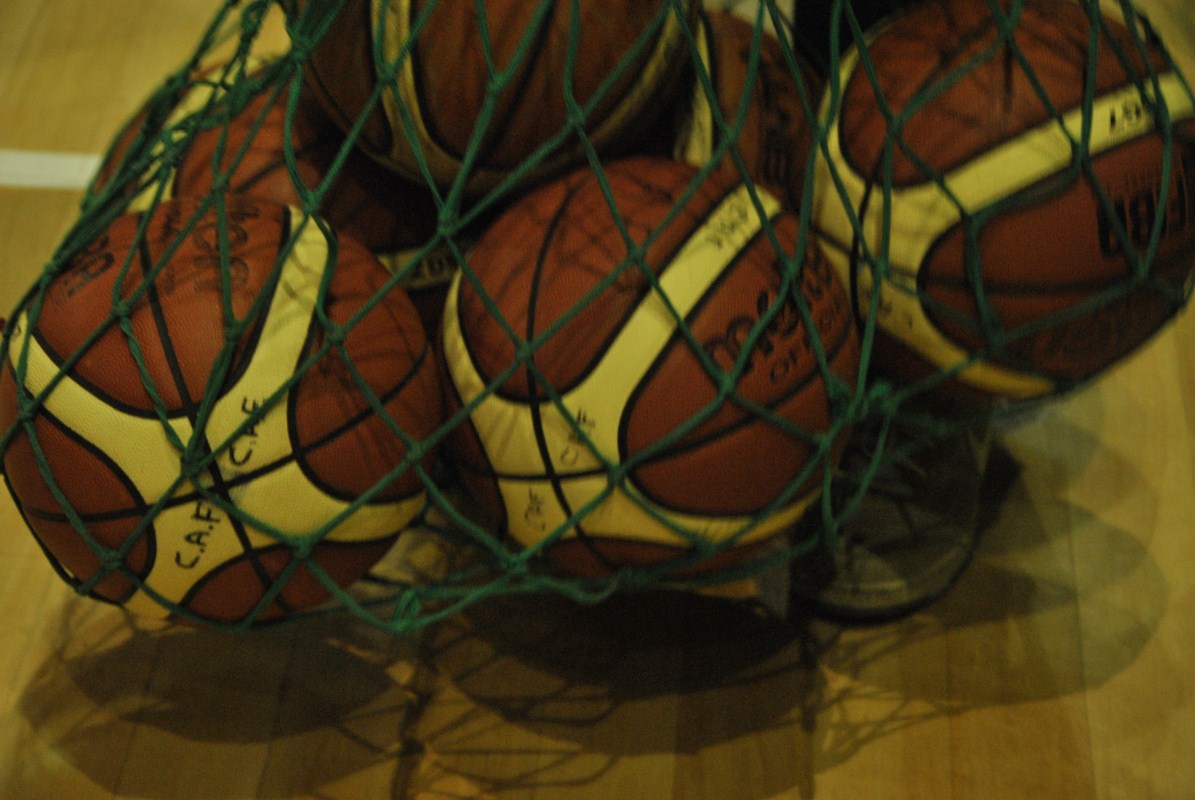This is a close-up color photograph of a net bag holding a collection of basketballs, the kind typically found in a school gymnasium. The dark green netting, reminiscent of a Christmas tree hue, contains predominantly dark orange basketballs adorned with four broad white stripes around their circumference, converging in a cross pattern. Although there is text where the stripes meet, it is difficult to decipher due to the low resolution and the balls' varying orientations. The net bag of basketballs is resting on a classic gymnasium floor, characterized by mahogany-colored wooden planks running from the foreground to the background. There is a hint of white court markings in the top left corner of the image, partially visible. Additionally, a gray shoe, possibly a Nike sneaker, can be seen at the edge of the frame, suggesting the presence of an individual. The basketballs cast shadows on the floor, implying that there is overhead lighting illuminating the scene.